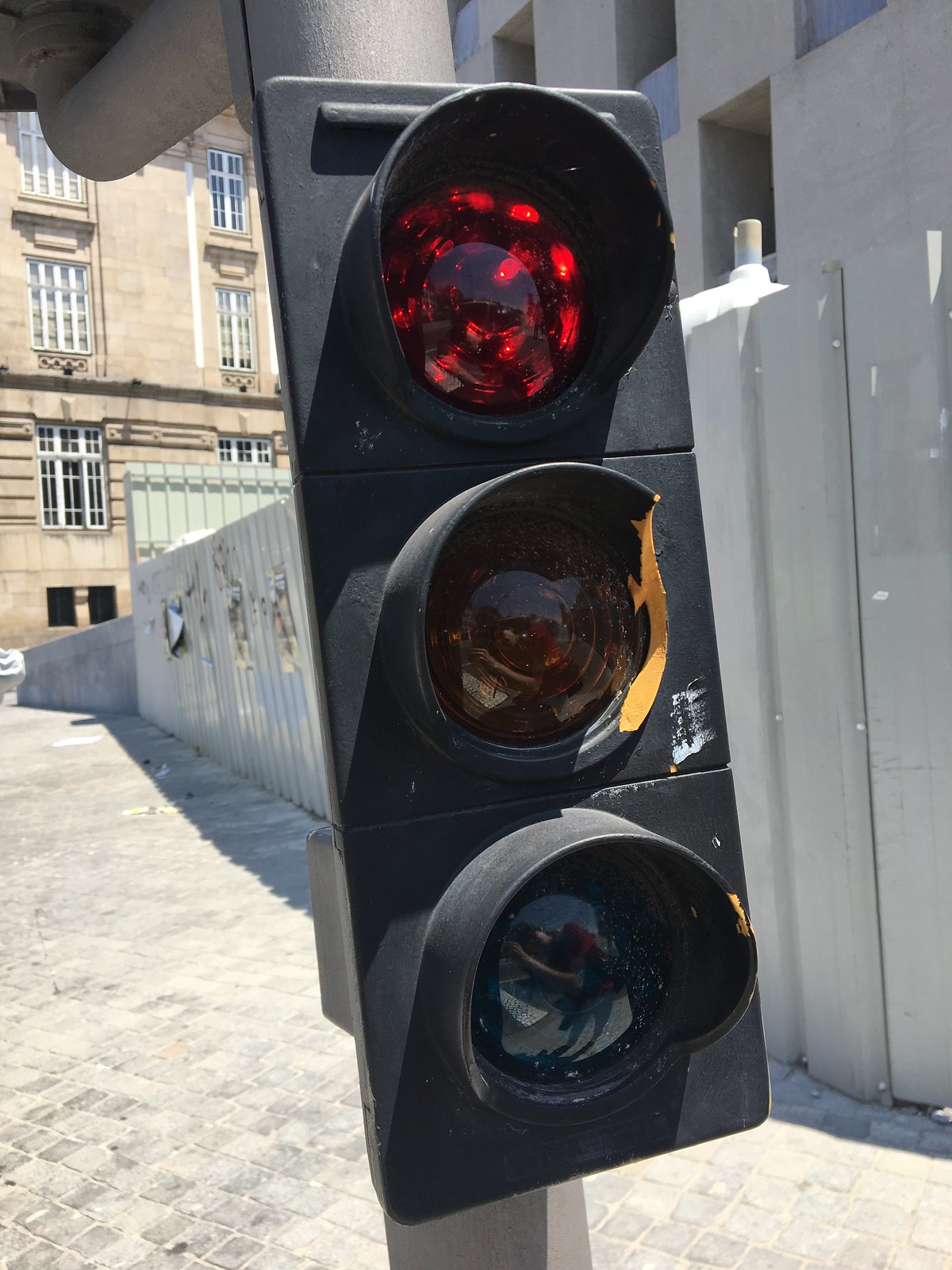In this close-up photograph taken in broad daylight, a traffic light is prominently featured at eye level, mounted on a gray pole. The traffic light's red signal is illuminated, while the yellow and green lights remain unlit. The traffic light itself shows signs of wear, with chipped plastic guards around the LED bulbs and faded paint. Behind the traffic light, a diverse backdrop unfolds including a white fence, a long white-grey wall adorned with graffiti, and a stone pavement. Further in the background, a green building can be seen, resembling a small-town American courthouse, characterized by a light brown facade with white-bordered windows. The scene is detailed and textured, with the sun casting its midday light over the various elements.